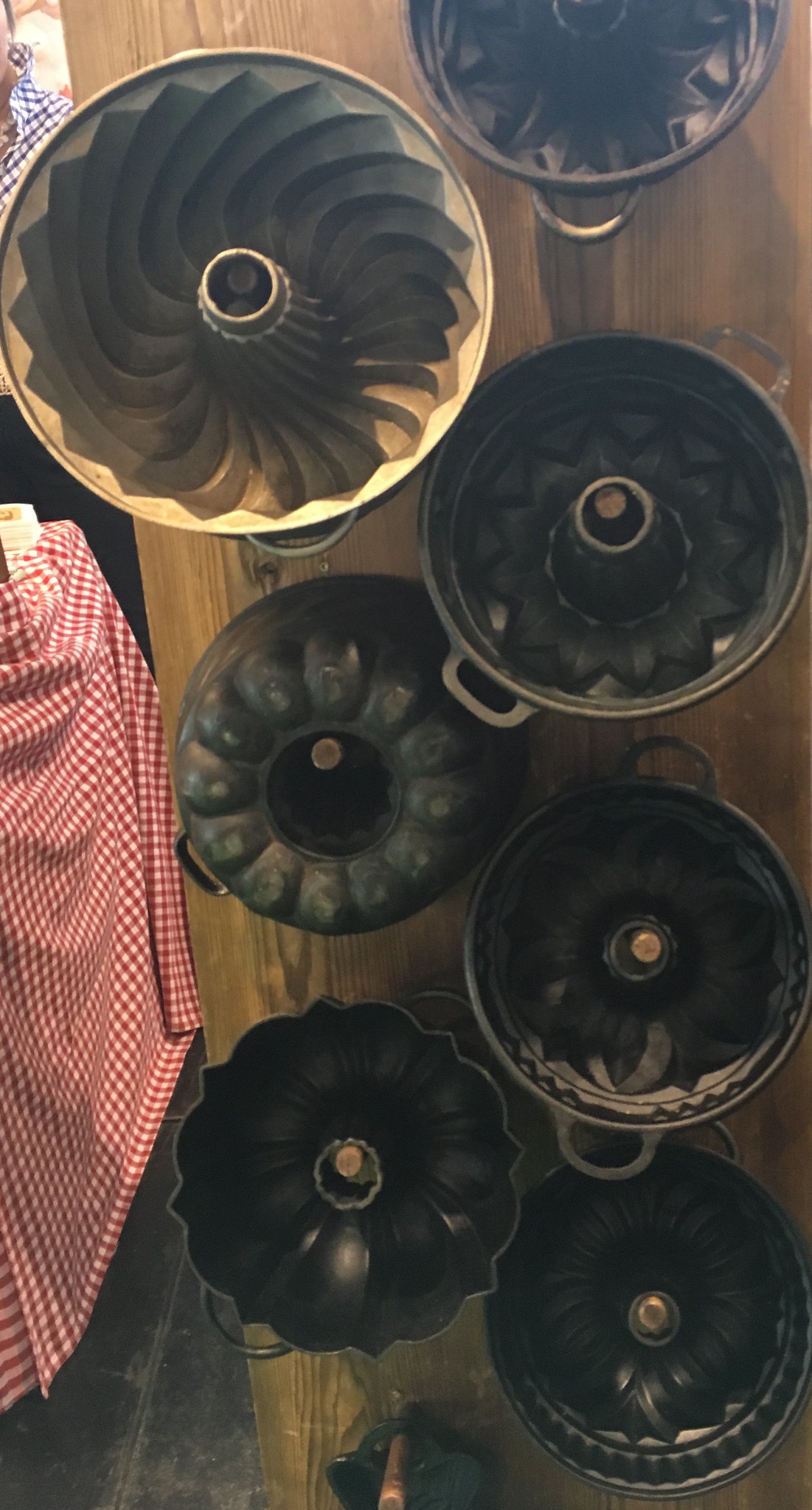This colored photograph features an aerial view of a large set of eight Bundt cake pans arranged together on a light, somewhat unfinished wooden table. Seven of the pans are positioned upright, ready for batter, showcasing their beautiful scalloping and circular shapes with central cylinders ideal for making pound cakes, while one pan is inverted, revealing its bottom. The pans display a range of wear, suggesting they have been well-used. They vary in material and color—some are bronze-colored metal, two are notably darker nearing black, and one is a light brown or tan silicon pan. Some pans have handles whereas others do not. In the background, a table with a red and white checkerboard tablecloth adds a splash of color, enhancing the rustic charm of the scene. Wooden pegs are visible, indicating a storage or display aspect to the arrangement.